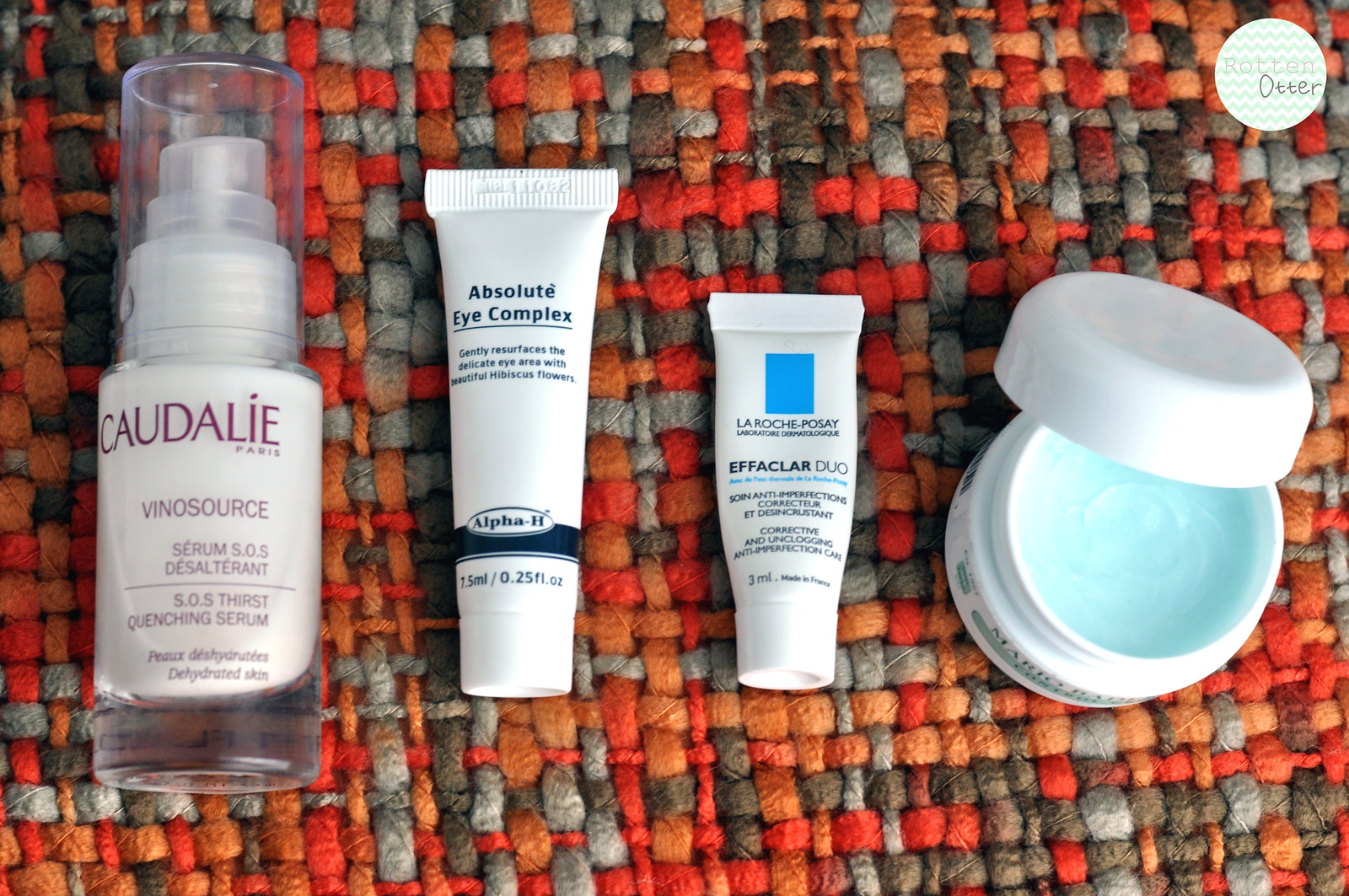The image showcases a collection of four cosmetic products laid evenly across a colorful, woven placemat. The placemat features an intricate weave of orange, red, and gray hues. Positioned in the upper right corner of the image is a small, white circle adorned with gray squiggles and the faint, gray text "rotten otter."

Occupying the bulk of the image, the four cosmetic items are meticulously arranged from left to right:

1. **Caudalie Vinoperfect Serum**: A pump bottle equipped with a transparent plastic cap, prominently displaying the brand name "Caudalie" and the product name "Vinoperfect Serum."
   
2. **Absolute Eye Complex**: A sleek, white tube with bold, black lettering identifying the product as the "Absolute Eye Complex."
   
3. **La Roche-Posay Effaclar Duo**: A squat white tube highlighted by a blue rectangle near the dispensing end, and black text that reads "La Roche-Posay Effaclar Duo."
   
4. **Transparent Gel Container**: A short, cylindrical white plastic container with a white lid that is slightly set back, revealing the transparent gel inside.

The careful arrangement and detailed depiction of each product against the vibrant woven backdrop create a visually appealing and informative composition.